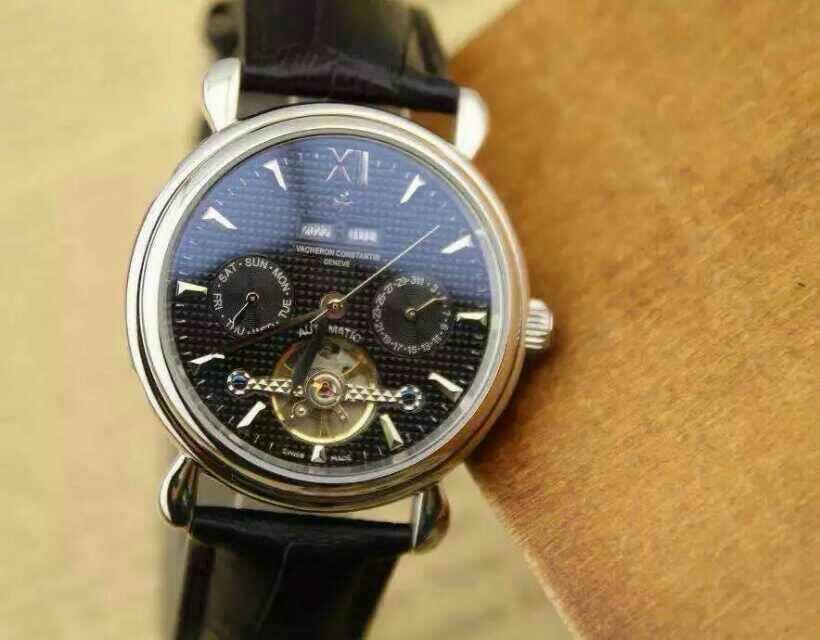A close-up photograph captures a sophisticated wristwatch resting on the edge of a wooden table. The watch boasts a glass face encased in a gold rim, set against a black, ribbed-texture background that exudes elegance. Prominently displayed at the 12 o'clock position, the only numeral on the dial is a Roman numeral XII, which adds a classic touch. The timepiece features a silver second hand and two black hour and minute hands, which subtly blend into the dark backdrop, making them somewhat challenging to read. Enhancing the watch's luxurious appeal, the band is black and shiny. Two smaller sub-dials gracefully provide additional information, indicating the day of the week and the day of the month. Positioned at the bottom center of the face, a larger gold teeter-totter mechanism adds a dynamic and intricate element to the overall design.